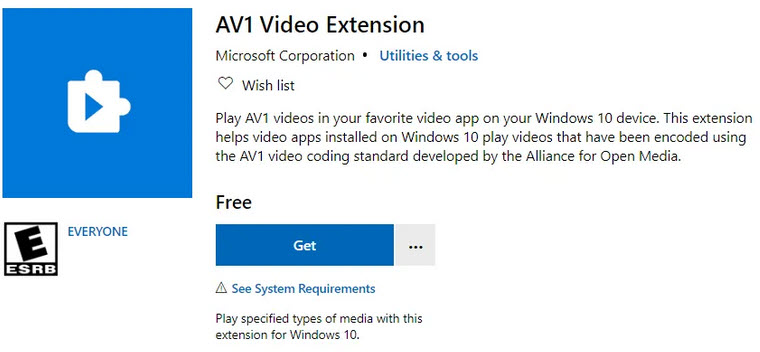**Screenshot Description: AV1 Video Extension Overview**

The screenshot captures an interface for installing the "AV1 Video Extension" on a computer. The left side of the image features a blue icon displaying a white puzzle piece at its center, with a blue play button symbol cleverly integrated within the puzzle piece.

At the top center of the interface, bold text reads "AV1 Video Extension." Directly below this, the text specifies the category as "Corporation Utilities and Tools." A heart icon underneath the text allows users to add the extension to their Wishlist.

The main description below these headers informs users that the extension enables video apps on Windows 10 to play videos encoded with the AV1 video coding standard, developed by the Alliance for Open Media. The extension is available for free, indicated by the word "Free" prominently displayed below the description. A large blue "Get" button encourages users to download the extension.

Additional information includes a link to "See System Requirements," ensuring users can verify compatibility before installation. The extension promises to "play specified types of media with this extension for Windows 10," emphasizing its role in enhancing media playback capabilities on the platform.